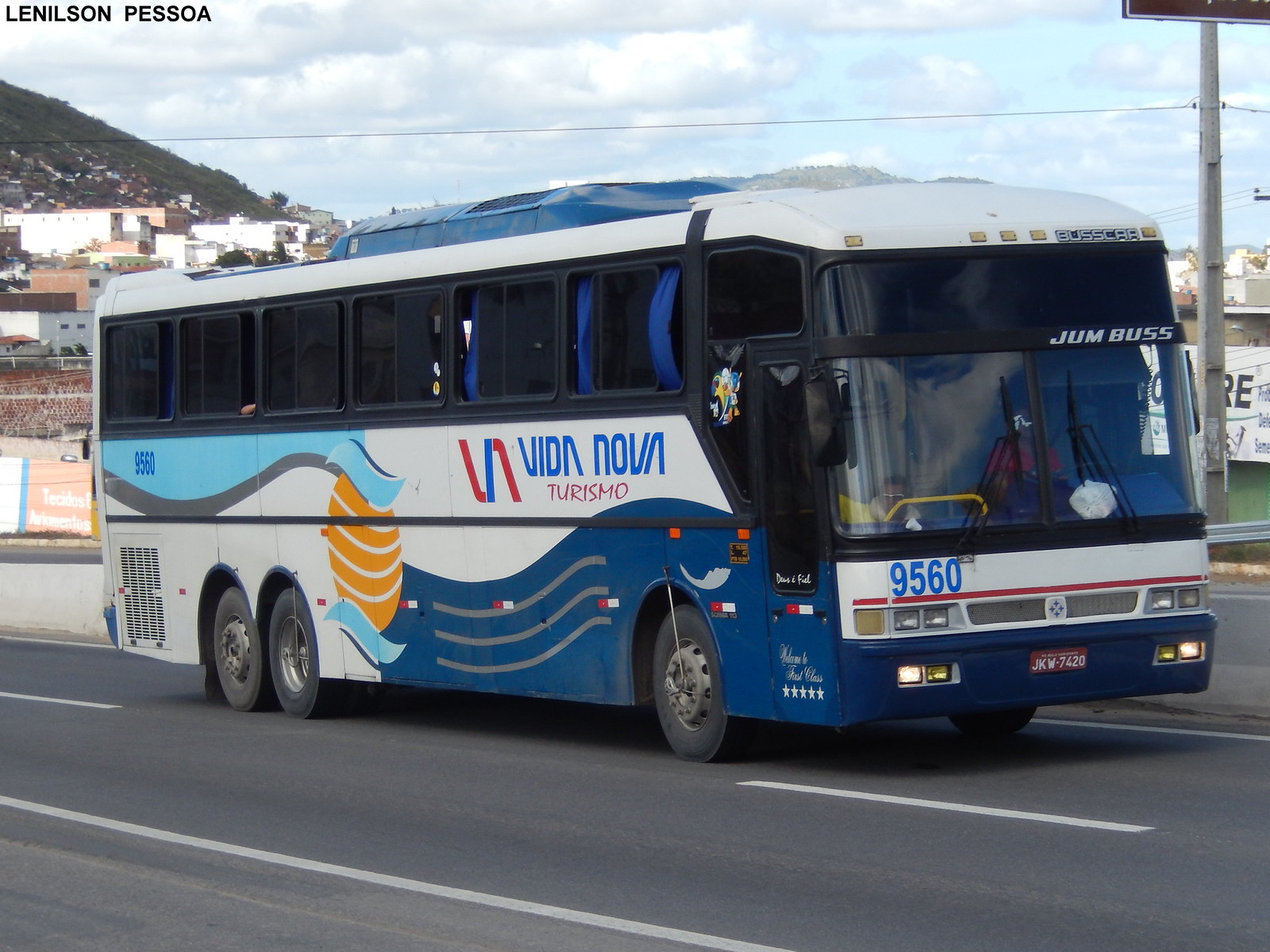The photograph depicts a long-distance tourism bus traveling on a well-maintained road. Captured from a 45-degree angle, the elevated passenger section sits above the bus’s sizeable lower luggage compartment. The bus has "Jump Bus" displayed above the driver’s window. The scenic background includes the side of a hill adorned with white buildings, a stretch of the sky, and the top of another hill in the distance.